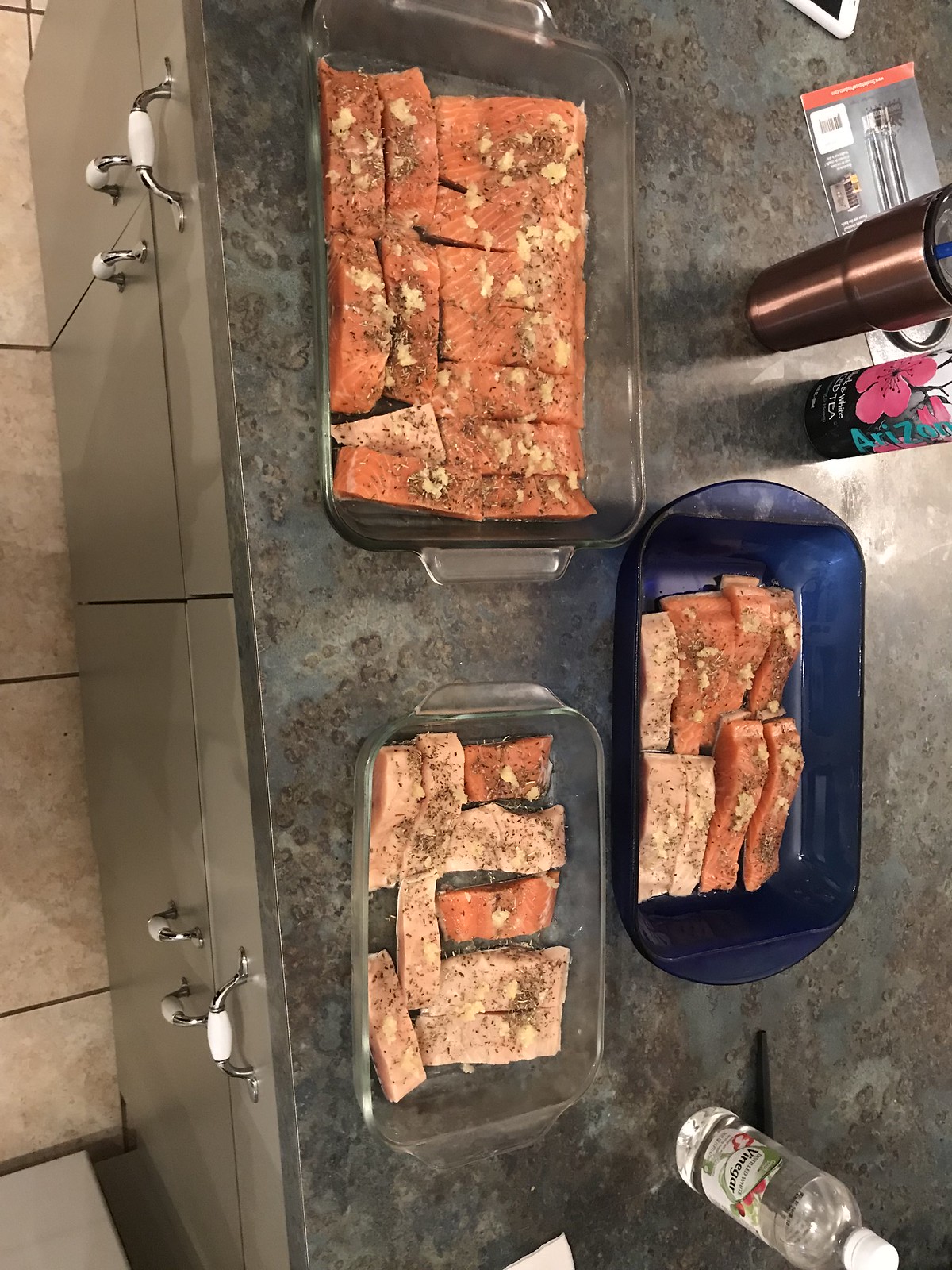This image captures an overhead view of a professional kitchen countertop, suggesting an environment where meal preparation is actively taking place. The countertop, possibly slate-colored, is adorned with three large glass trays filled with salmon fillets. The salmon showcases two shades of pink—light and medium—and is meticulously seasoned with spices and garlic. Accompanying the trays on the countertop are a few other items: a clear bottle labeled as white vinegar with a white cap, a copper-colored tumbler with a handle, and a can of Arizona tea featuring a hibiscus flower with blue writing. Below the countertop, there are visible handles and drawers, hinting at a well-organized kitchen setup. The floor beneath the counter has a tan-patterned, pinkish-brown tile, providing a warm contrast to the kitchen’s functional surfaces. The image also appears to be taken sideways, adding a unique perspective to the scene.